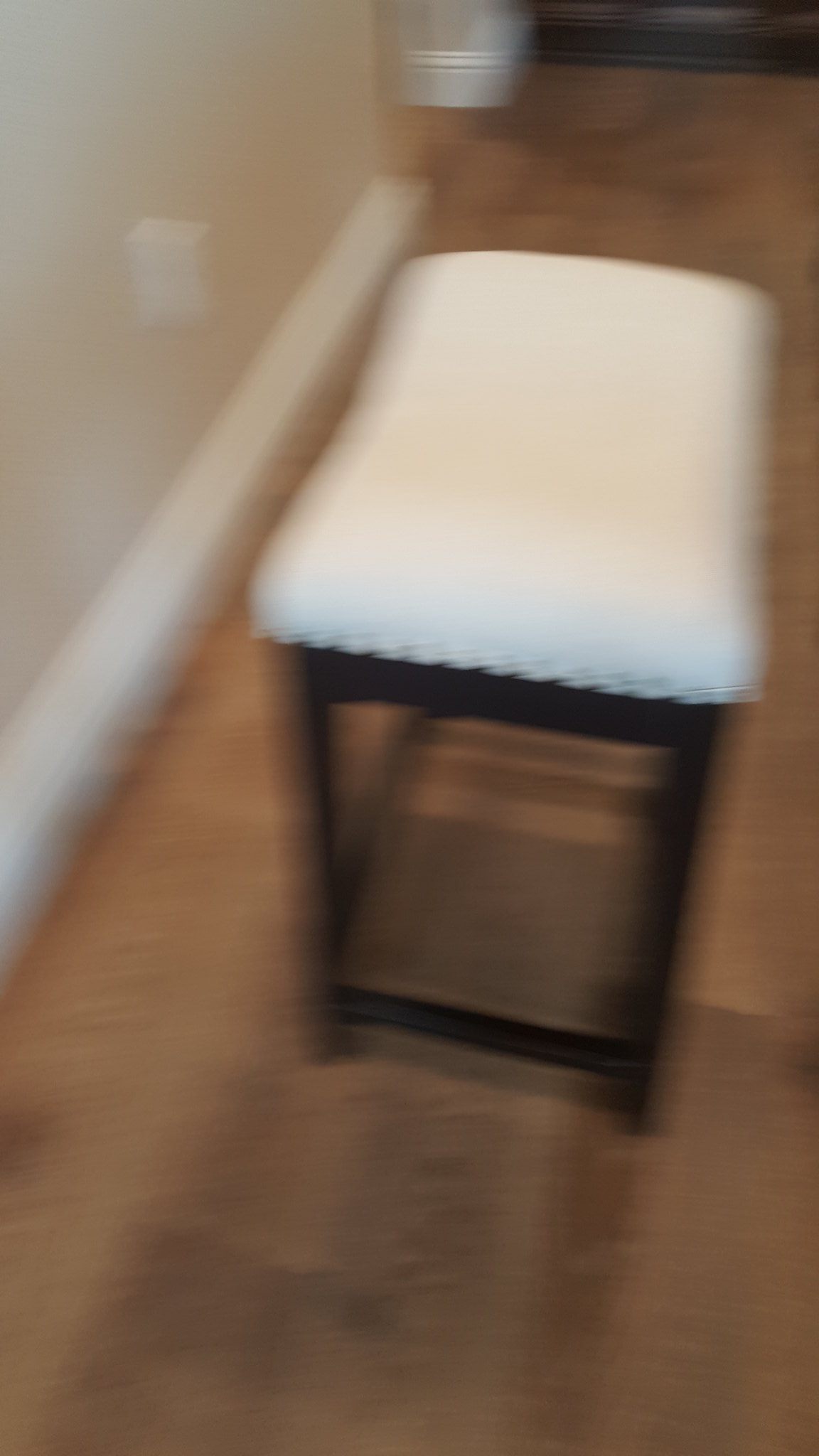In the photograph, a stool occupies the central space of a somewhat blurry hallway. The stool, distinguished by its black legs, features a white cushioned top and a shelf beneath the seat. The hallway is lined with a wall runner and brown carpeting, which appears freshly vacuumed given the visible color variations. To the right side of the stool, an electrical outlet can be identified on the wall. As the hallway extends, it turns to the left, suggesting a continuation of the corridor. The backdrop shows a brown wall, with no other objects situated around the stool, emphasizing its solitary presence.